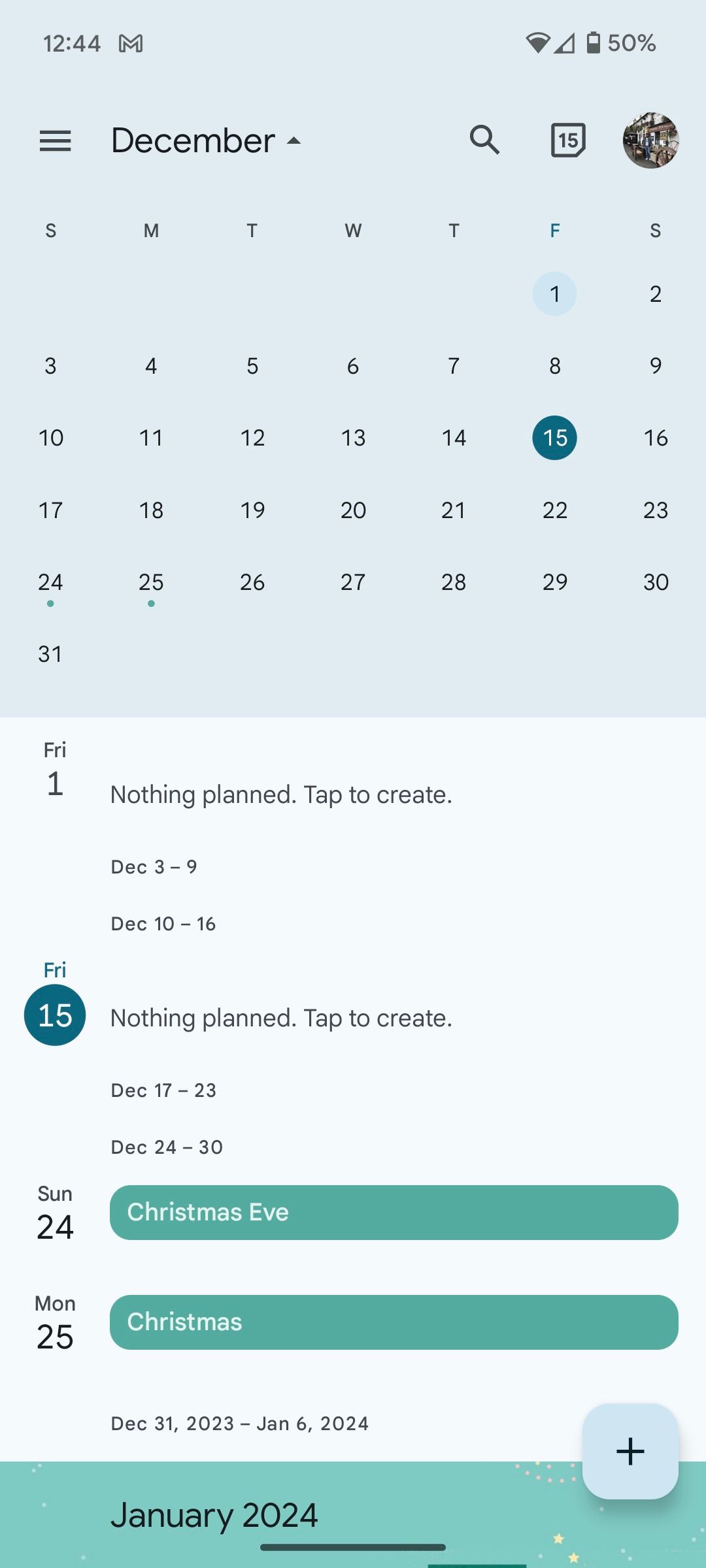The image depicts a screenshot of a mobile device's calendar application, showcasing the user's December agenda. At the top, there's a monthly view of December, with dates clearly displayed. Notably, the 24th and 25th are marked with dots, signifying scheduled events—Christmas Eve and Christmas Day, respectively. Below this monthly view, there is an agenda section. Today's date is identified as Friday, December 1st, with a note that nothing is planned and an option to tap and create an event.

The agenda view is broken down into weeks, with the periods from December 3rd to 9th and December 10th to 16th indicating no scheduled events. However, on the calendar above, Friday the 15th is highlighted, which also appears in the agenda view with "nothing planned, tap to create." As the weeks progress, the agenda lists Sunday the 24th as having an all-day event for Christmas Eve, followed by Monday the 25th for Christmas, also marked as an all-day event. 

At the bottom of the screen, a green bar features a prompt for "January 2024," accompanied by a plus icon for creating new events. The interface suggests it is likely an Android device utilizing the Material You design language, although it does not appear to be the stock Android calendar application.